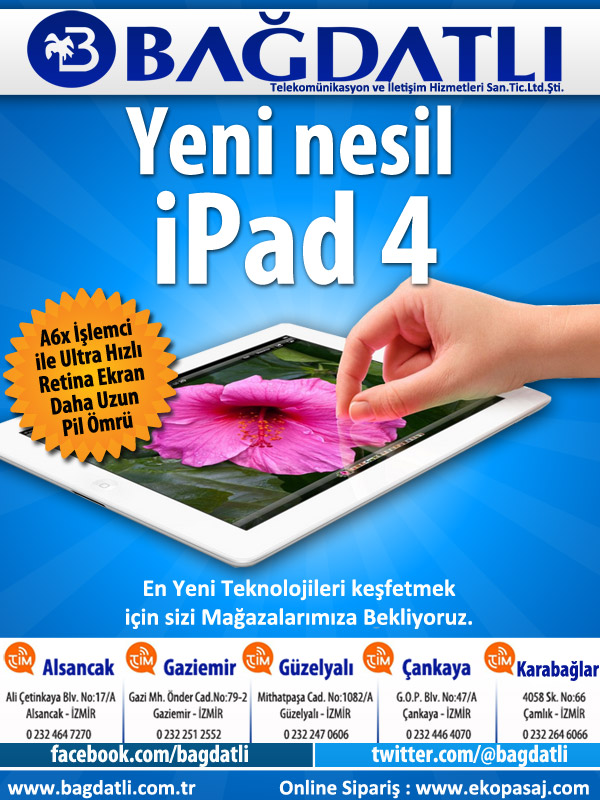This image is an advertisement for the iPad 4, likely in Turkish. The majority of the background is blue, creating a vibrant setting for the ad. At the top, a white rectangular banner features blue lettering, with "B-A-G-D-A-T-L-I" prominently displayed. Below this, the ad transitions to a deep blue background where white text spells out "Y-E-N-I-N-E-S-I-L" followed by "iPad 4". Dominating the center of the image, the iPad is presented in a three-quarter view, slightly tilted on its side. A person's hand with light skin tone is reaching in from the right, pinching the top of the iPad screen that displays a striking image of a bloomed pink hibiscus flower with green leaves. To the left of the iPad, a circular overlay with black lettering and a zigzag edge stands out. The bottom part of the ad includes more blue text that is too extensive to fully capture. The advertisement also showcases social media icons and addresses, with clear calls to action to connect on Facebook and Twitter, along with a blue rectangle at the very bottom containing additional text, potentially a website URL.